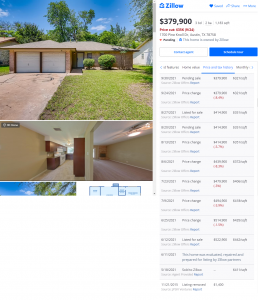In this image, we see a property listing from Zillow, highlighting a house priced at $379,900. Although some details are difficult to read due to poor image quality, the photograph of the house reveals a well-maintained exterior. The house features two garage doors and a driveway, surrounded by a lush lawn adorned with vibrant flowers. Tall trees can be seen in the background, adding a touch of natural beauty to the setting. The bottom part of the image showcases the interior of the house, displaying a cozy, well-decorated space. The interior decor includes clothes and accessories in shades of blue, green, white, and brown, contributing to a warm and inviting atmosphere.